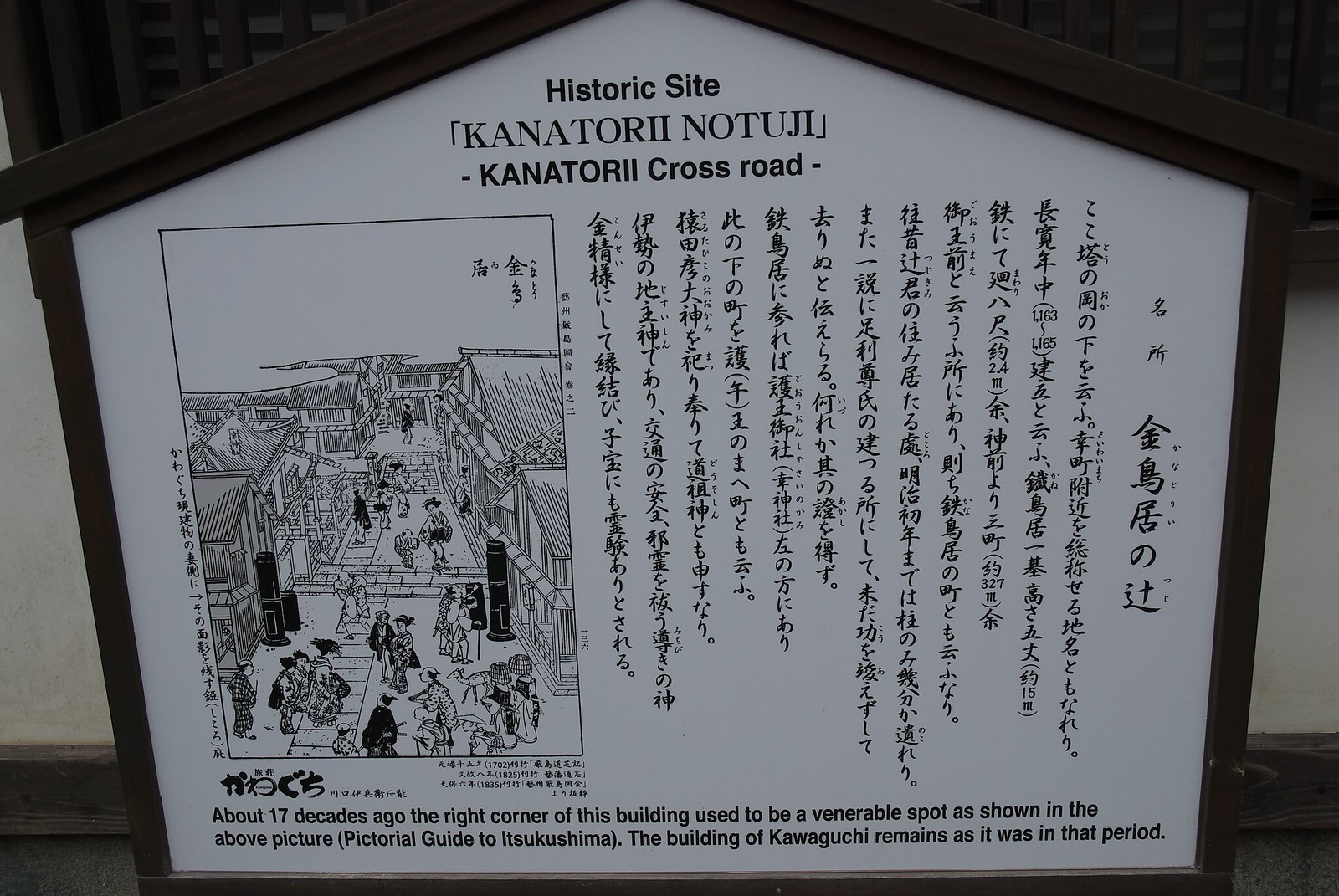In the image, we see a stylized house-shaped signboard with black borders and a white background, standing in front of a memorial which features a wall that is white at the bottom and black at the top. The signboard prominently displays the heading "Historic Site Kanatori Notoji Kanatori Crossroad" at the top. On the left side of the signboard, there is a black and white hand-drawn illustration, resembling a woodblock print, depicting a bustling marketplace scene in Japan, with people of both genders and some animals walking down a street flanked by shops and staircases. The illustration is contained within a box and is captioned in Japanese. To the right of the illustration, there is a significant amount of text in Japanese, with numbers like 32711631 and 1165 scattered throughout. At the bottom of the signboard, a footnote reads, "About 17 decades ago, the right corner of this building used to be a venerable spot as shown in the above picture (Pictorial Guide to Itsukushima). The building of Kawaguchi remains as it was in that period."